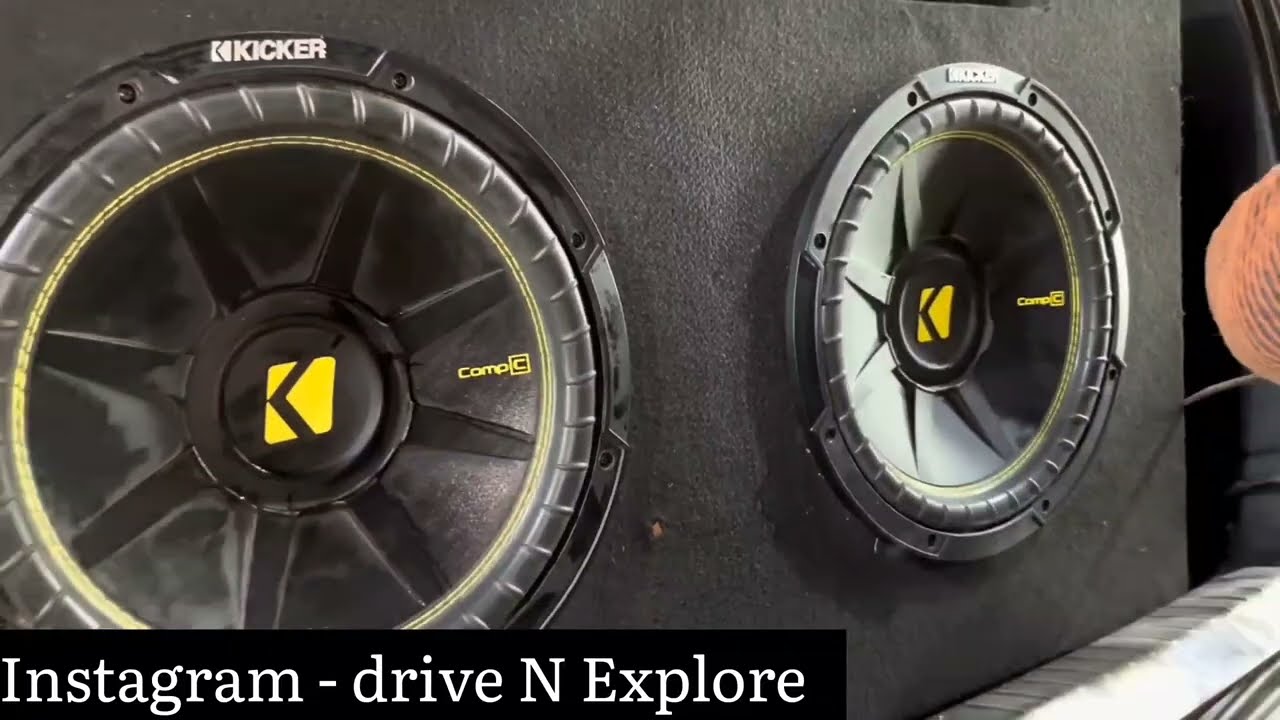The photograph showcases a close-up view of a black speaker, set against a slightly textured, fabric-like surface with the device tilted slightly backward to the side. Dominating the left side of the image are two large circular subwoofers recessed into the surface, each featuring intricate design elements. The topmost circle prominently displays "KICKER" in white text. Below this, a sequence of nested circles includes a main black circle with notched edges, a yellow circle, and a central section resembling bicycle spokes radiating towards a black center with an emblem. The emblem consists of a predominantly yellow triangle with a black arrow pointing left. On the right side of each subwoofer, the word "Comp" appears, followed by a square with the letter "C" inside it.

Additionally, a touch of orange, possibly part of someone's clothing, is visible on the far right, resembling an elbow sticking through. At the bottom left of the image, a black rectangular bar features the text "Instagram - Drive in Explore" in white. The overall image captures the detailed branding and design intricacies of the speaker, emphasizing its bold geometric patterns and textured surface.